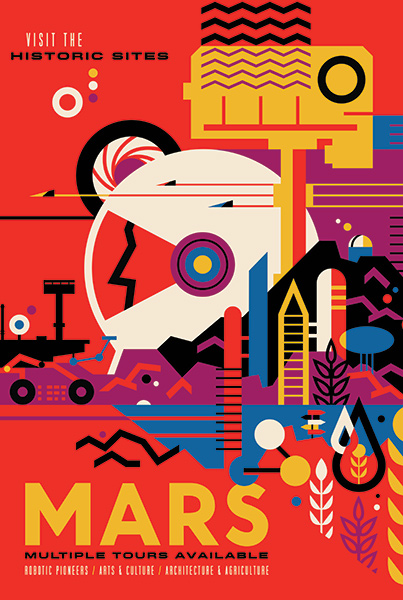The image is a vibrant and colorful poster set against a rich red background, prominently featuring the text "Visit the Historic Sites" at the top. The main focus is on the word "MARS," boldly displayed at the bottom, accompanied by the phrase "multiple tours available." The poster lists "Robotic pioneers, arts and culture, architecture, and agriculture" as highlights of the tours.

Central to the design, there's a figure in a stark white helmet adorned with a multicolored earpiece, featuring hues of purple, yellow, and blue. The poster is adorned with various intricate designs, including what appear to be plants, water, robotic elements, and possibly cannabis. Additionally, there are other images, including one that resembles a car and another that looks like silos, contributing to the theme of exploration and history. The text on the poster is in diverse colors—white, black, and gold—adding to its eye-catching appeal.